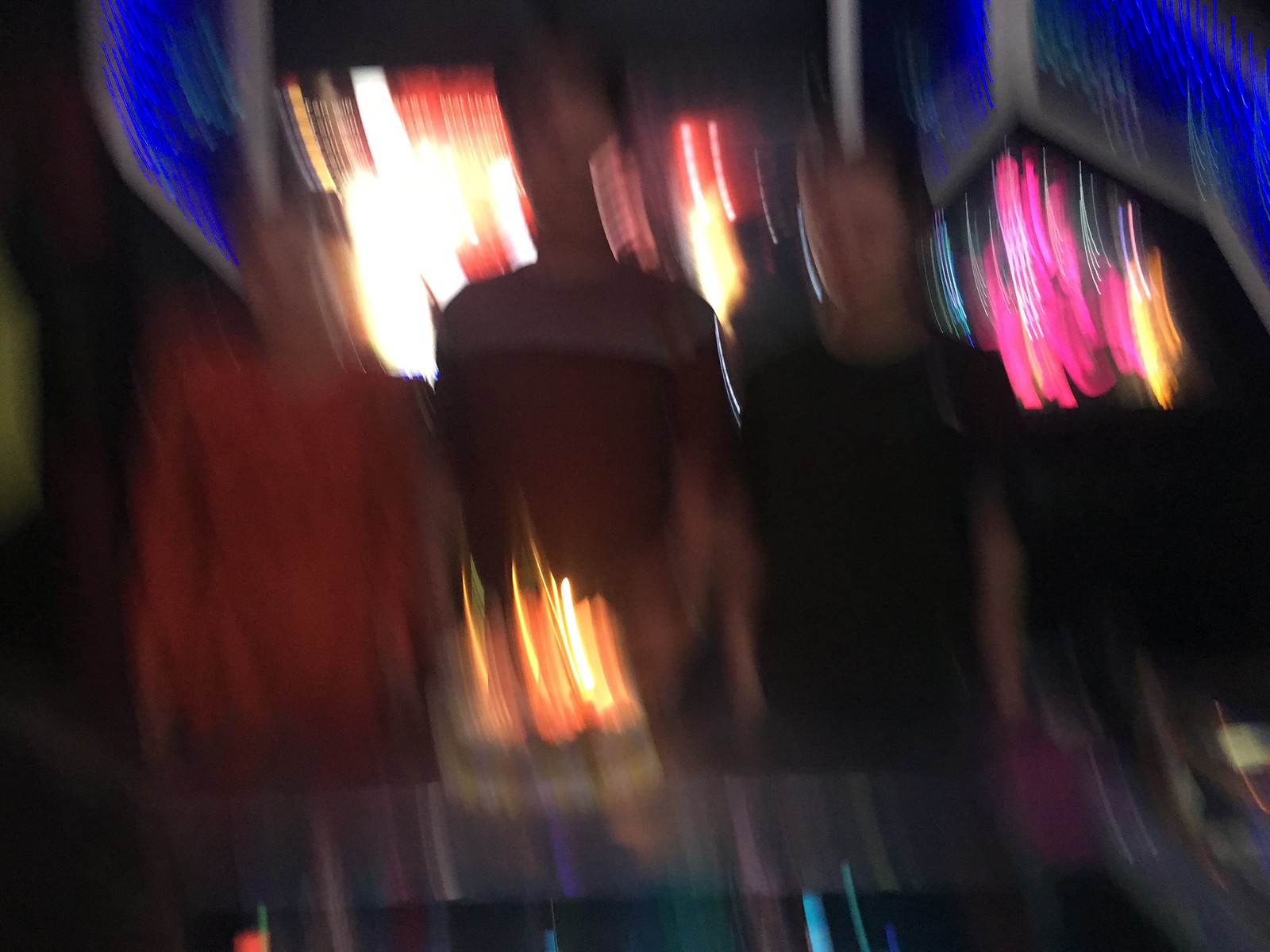This heavily blurred night-time image features three adults standing indoors, likely at a bustling amusement venue or popular arcade restaurant such as Dave and Buster's. They are positioned in front of a celebratory cake, which could be for a birthday or another event. In the background, unfocused city-like lights create streaks of royal blue, white, yellow, pink, and golden hues, adding to the disoriented look. The person on the left appears to have long blonde hair and is possibly wearing a blouse, suggesting they might be female. The two individuals on the right, potentially males, have shorter hair. The colors of their attire seem to range from orange to red to black, although the blurriness makes specifics hard to discern. The photo overall suffers from significant motion blur, making finer details indistinguishable.